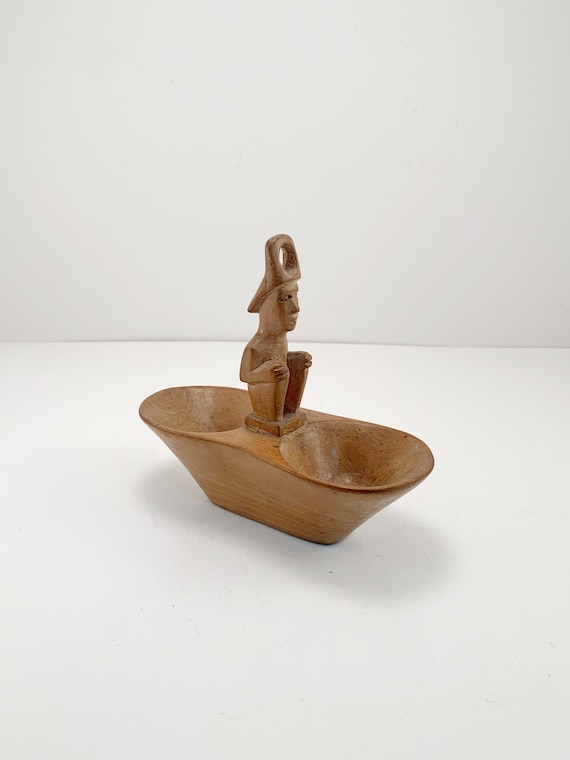The image depicts a light brown, wooden artifact, appearing as if it might be an ancient piece showcased in a museum. The object features a central oval section reminiscent of a small boat or a pair of conjoined bowls. Seated atop this structure is a carved wooden figure of a man in a squatting position, with neutral facial features and closed eyes. He has his knees drawn up in front of him and his hands resting on them. The figure is adorned with a hat that has a hole at its top, possibly suggesting it serves as a handle or holder. The background is entirely white, with the object centrally positioned, likely resting on a similarly white surface. The overall image emphasizes the contrast between the crafted wooden artifact and its stark, clean background.